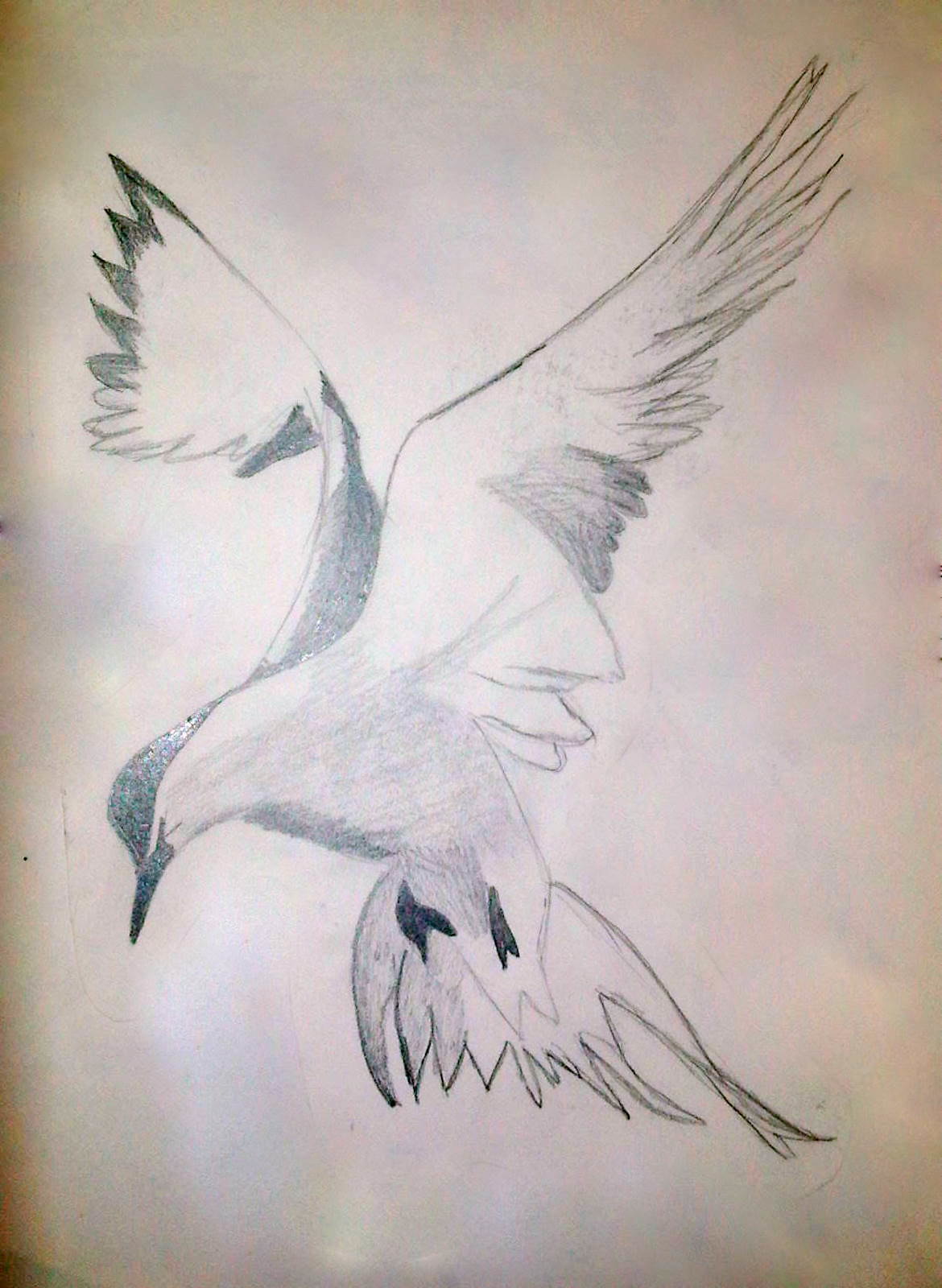This is a close-up photograph of a pencil drawing on a white sheet of paper, featuring a bird in mid-flight. The bird, resembling a tern, possesses long, ornate wings with a substantial wingspan, creating a forked Y-shape above its body. Its head, adorned with a black cap, is bowed slightly downward as it faces the left in a three-quarter profile, its black beak visible. Its underside is prominently displayed, with two black feet hanging beneath it, and a fan-like tail stretching down and to the right.

The drawing employs a black and white style, with the bird’s wings shaded in a grayish-white hue, and the tips and upper portions darkened for emphasis. The background has been lightly shaded and blurred, adding texture and depth to the illustration. The image is detailed, capturing the texture of the graphite pencil, with light reflecting off several areas, suggesting the use of a camera flash. Despite its intricacy, the drawing, which lacks any text, signature, or markings, appears to be well-crafted but not professional. The overall lighting is somewhat dark, further highlighting the pencil's tonal contrasts.